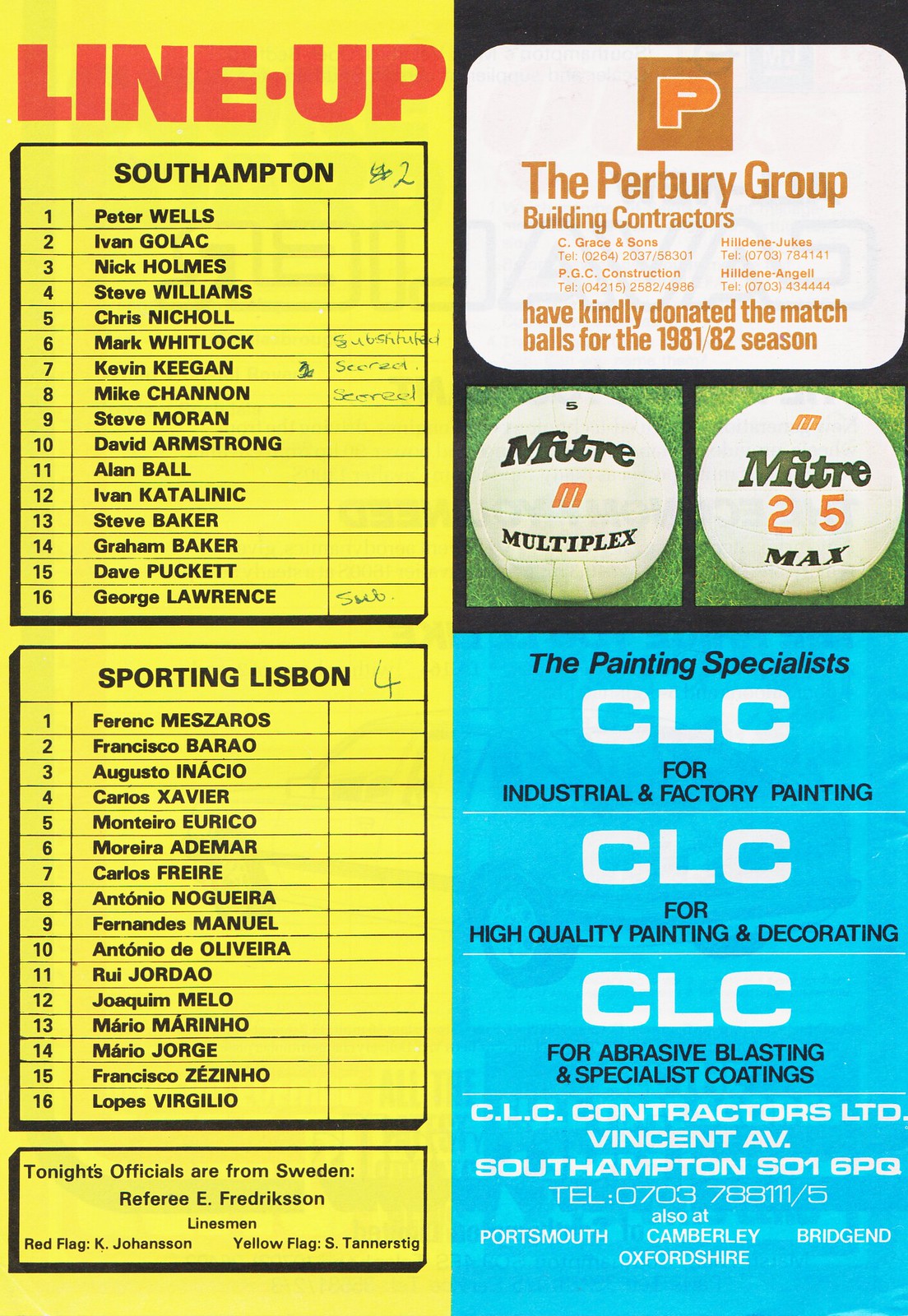The image is a scan of a football club program from England, highlighting a match between Southampton and Sporting Lisbon. The left side of the image is dominated by a large yellow section with black text labeled "Lineup" in bold red letters. The Southampton lineup includes names such as Peter Wells, Ivan Golak, Nick Holmes, and Kevin Keegan, among others. Notes in green pen are visible next to some names. Below this, it lists the match officials from Sweden: referee E. Fredrickson, linesmen Kay Johansson (red flag), and S. Tennerstig (yellow flag).

On the right side, there is a white box with brown text indicating that "The Perbury Group, building contractors, have kindly donated the match balls for the 1981-82 season." Below this are images of two Mitre Multiplex soccer balls. Further down is a blue box with alternating black and white text promoting CLC Contractors Limited for various painting and coating services. Their contact details are provided, including an address at Vincent Avenue, Southampton, and a telephone number (0703-788-111). Other locations listed include Portsmouth, Camberley, Bridgend, and Oxfordshire.